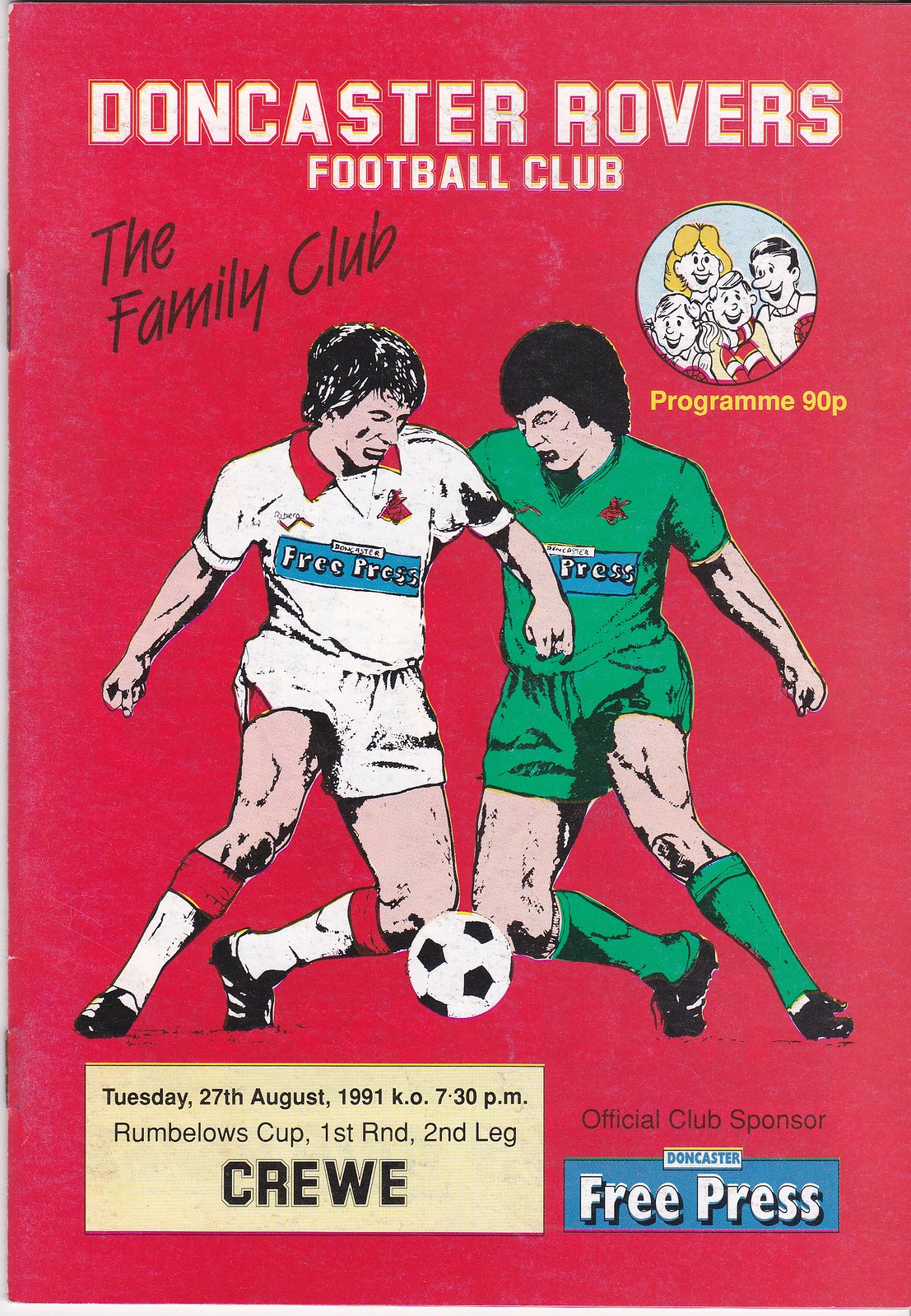This image appears to be an advertisement for a Doncaster Rovers Football Club game day program from the early 1990s, specifically from Tuesday, 27th August 1991. The cover has a bright red background with white text at the top that reads "Doncaster Rovers Football Club" and black text beneath that reads "The Family Club." In the center, there is a large hand-drawn illustration of two football players competing for a soccer ball. The player on the left is wearing a white uniform with red accents, including red and white socks, while the player on the right is in a dark green uniform. Both players are depicted with white skin, and the player on the right has dark hair.

Above this central illustration, there is a circular graphic showing a family—a man, a woman, and two children (a boy and a girl)—all dressed in red and white, with yellow text underneath that reads "Program 90P." The bottom left corner of the cover features a yellow box with black text providing details about the match: "Tuesday 27th August 1991 kickoff 7:30 p.m. Rumblo's Comp first round second leg Crewe." In the bottom right corner, a text box states "official club sponsor Doncaster Free Press." The jerseys of the players also display a symbol or logo that includes the name "Doncaster", with a blue rectangle that says "Free Press" inside it.